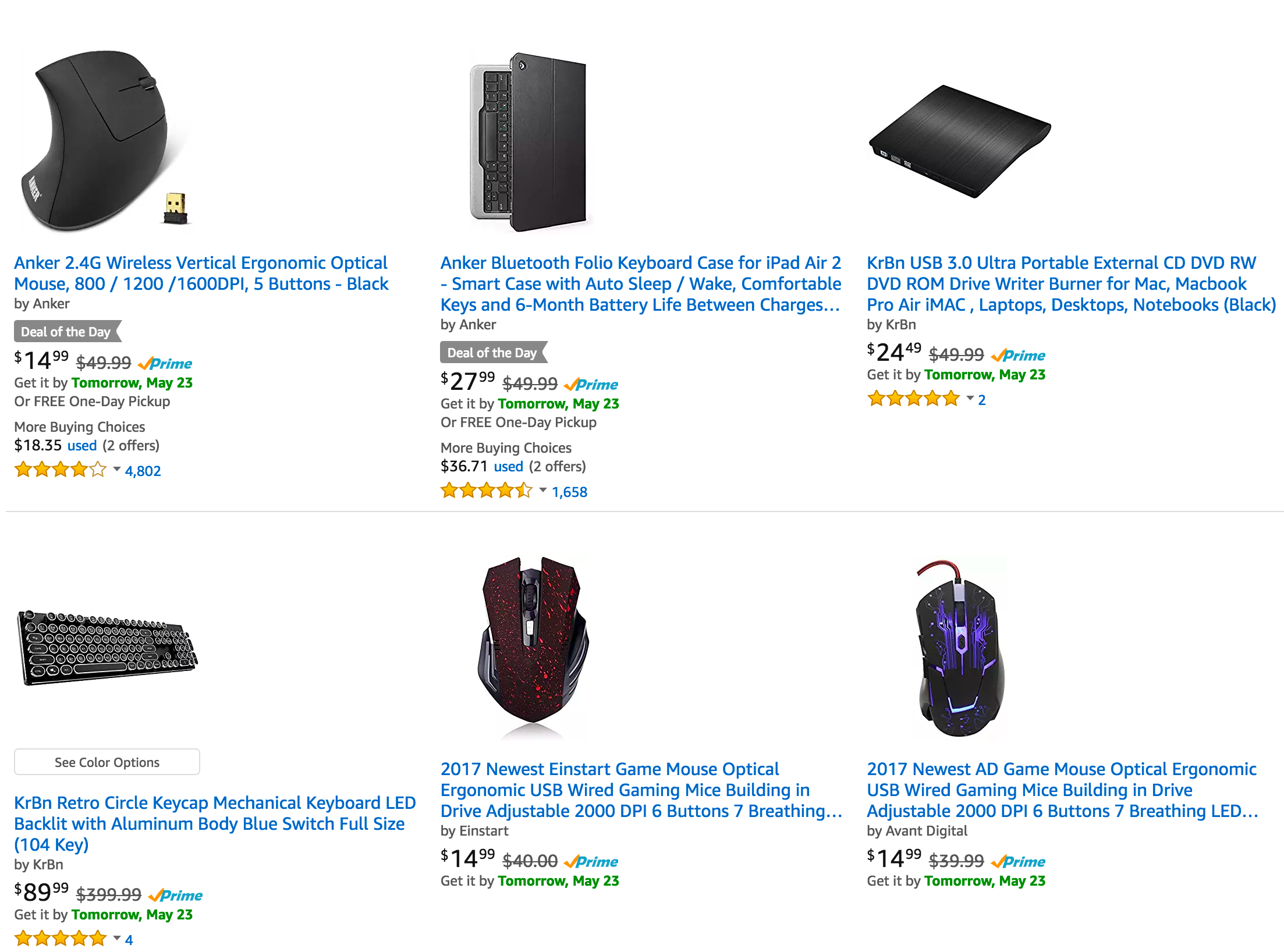Here's a cleaned-up and detailed caption:

---

**Amazon Product Listings:**

1. **Anker 2.4G Wireless Vertical Ergonomic Optical Mouse**
   - A sleek vertical ergonomic mouse designed for comfort, featuring wireless connectivity.
   - **Price:** $14.99 (discounted from a higher price, as indicated by the crossed-out amount)
   - **Special Offer:** Labelled as "Deal of the Day" with a grey background and white text.
   - **Availability:** Eligible for Prime with a guaranteed delivery by tomorrow, May 23rd, or free one-day pickup.
   - **Seller:** Anker

2. **Anker Bluetooth Folio Keyboard Case**
   - A protective keyboard case designed for efficient typing and secure tablet holding.
   - Presented in a similar format with an image of the product followed by a clickable blue link with the product name and seller information.

3. **KRMB USB 3.0 Ultra Portable External CD Drive**
   - An external CD drive offering high-speed USB 3.0 connectivity, compact and great for on-the-go use.
   
4. **KRMB Retro Circle Keycap Mechanical Keyboard**
   - A visually appealing mechanical keyboard with retro-style circular keycaps designed for a nostalgic typing experience.

5. **2017 Newest Einstein Game Mode Optical Mouse**
   - An advanced gaming mouse from 2017, featuring optical sensors for precision gaming.

6. **2017 Newest AD Game Mouse Optical**
   - Another high-precision optical gaming mouse from 2017, available in striking colors like red and blue.

---

This refined caption provides a clear and organized description of each listed item with specific details on prices, special deals, and key features.